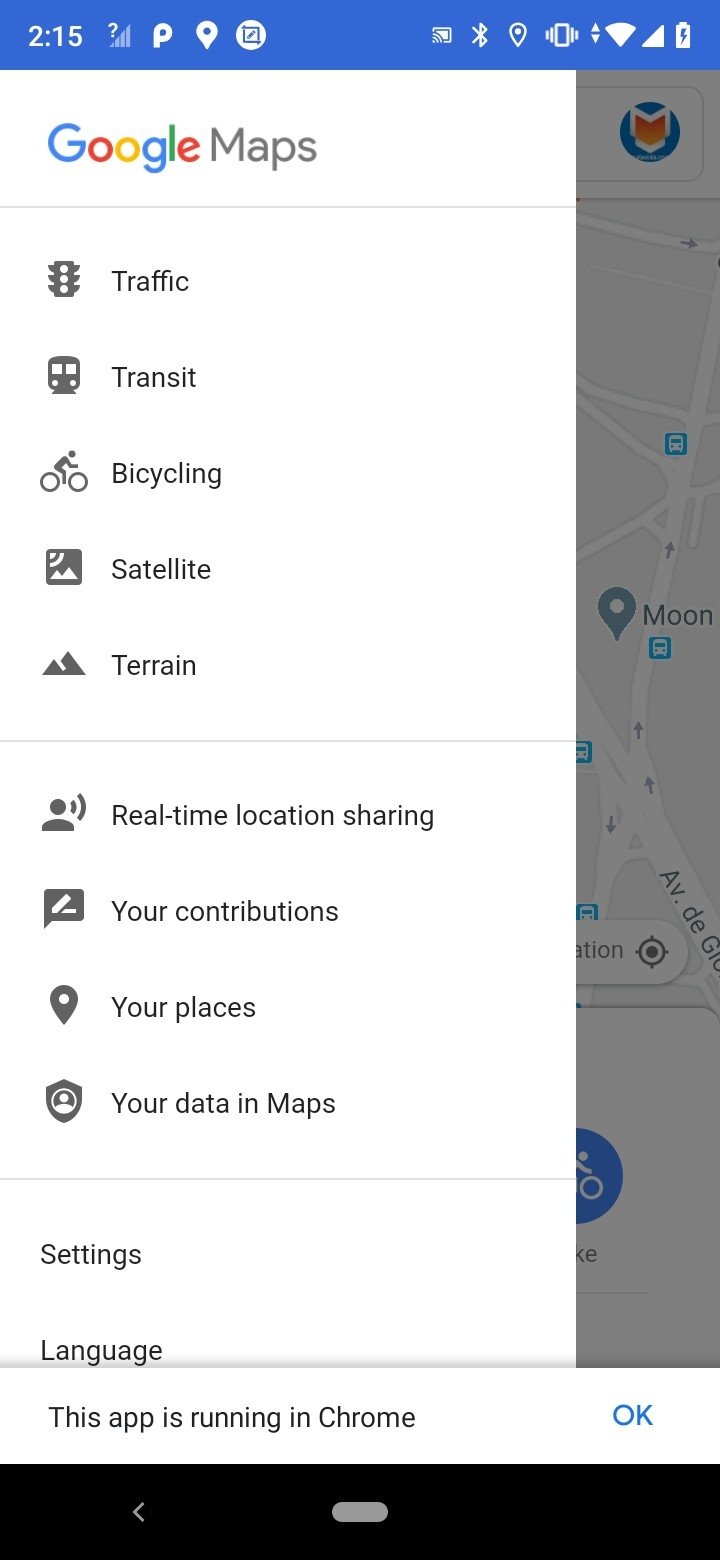The image displays a Google Maps interface with the menu fully expanded. The menu comprises several options, each accompanied by an icon for easy identification:

1. **Traffic**: Represented by a traffic light symbol.
2. **Transit**: Indicated with a train symbol.
3. **Bicycling**: Marked by a bicycle icon.
4. **Satellite**: Illustrated with an image of a satellite emitting rays.
5. **Terrain**: Denoted by a mountain symbol.

Further options include:
6. **Real-time location sharing**: Shown with an icon of a person with signal bars emanating from their head.
7. **Your Contributions**: Depicted with a chat box and a pen.
8. **Your Places**: Indicated with a place pin icon.
9. **Your Data in Maps**: Displayed with a shield containing a person icon.
10. **Settings**: Standard settings icon.
11. **Language**: Likely associated with a language selector icon.

Below these options, a bar states that "This app is running in Chrome," with an "OK" button to its right. Behind this expanded menu, a portion of the Google Maps interface is visible, displaying streets and typical map elements. 

In the top left corner of the interface, the time "2:15" is displayed alongside other various service icons. Thus, the image provides a comprehensive view of the Google Maps main screen with its menu and additional interface details.